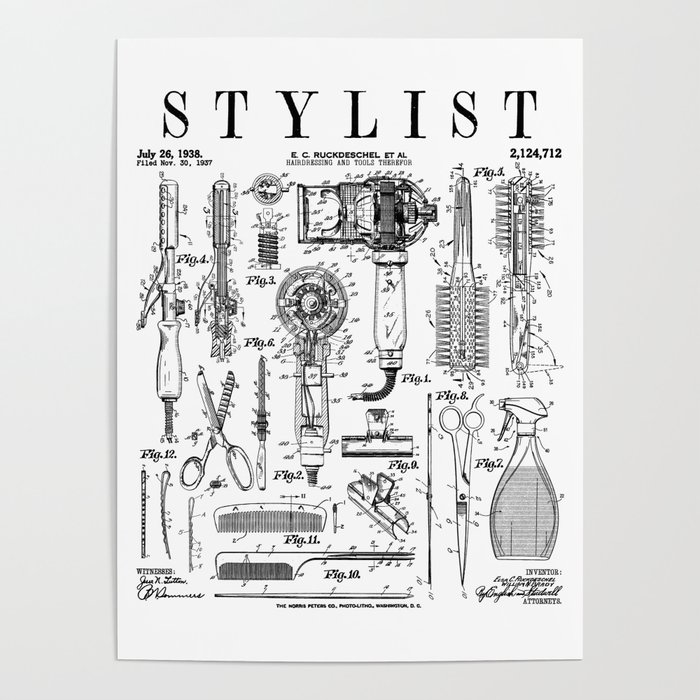The image depicts a black-and-white vintage publication page from July 26, 1938. At the top, the word "STYLIST" is prominently displayed in all caps, with "E.C. Ruckdeschel et al." and "HAIR DRESSING and TOOLS, THEREFORE" written below it. The page is filled with detailed illustrations of various hairstyling tools. On the top left, there is a curling iron with a smaller, detailed illustration next to it. Adjacent, on the top right, are two hairbrushes oriented in opposite directions. Below the brushes are two views of a blow dryer: one in profile and another showing the motor from the back. Scattered among these are images of hair clips, nail files, scissors, combs (including a rat-tail comb and a standard comb), a misting bottle, and what seem to be three different types of swabs. There are also a pair of shears and a sketch of a spray bottle. Each tool is meticulously labeled with blowout illustrations highlighting specific parts. The page, set against a light gray background, encapsulates a vintage black-and-white illustration style.